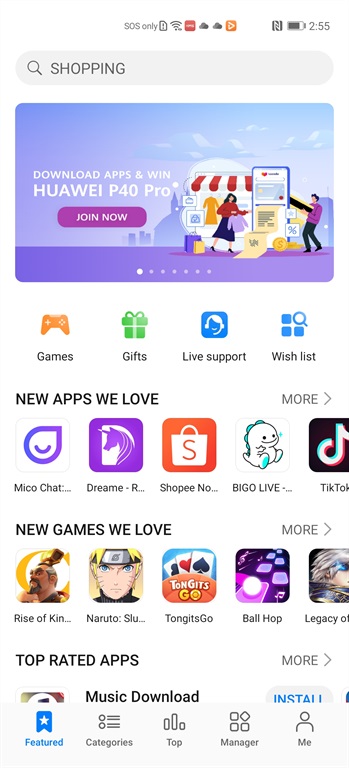A screenshot from a smartphone reveals a bustling app store interface. In the top-left corner, a search bar reads "shopping," while the top-right shows it is 2:55 PM with a nearly full battery at around 95%. Below, a promotional banner features an individual next to a food cart with the text "Download apps and win" followed by "Hawaii 4 or P40 Pro" and a prominent "Join Now" button.

Further down, icons for "Games," "Gifts," "Live Support," and "Wish List" are neatly arranged. The section titled "New Apps We Love" showcases a variety of apps including "MicoChat," "Dreamr," "Shopper-NO...", "BIGO Live," and "TikTok." Beneath this, "New Games We Love" leads into a category emphasizing trending game apps. At the very bottom, the "Top Rated Apps" section with clickable areas for further exploration completes the display.